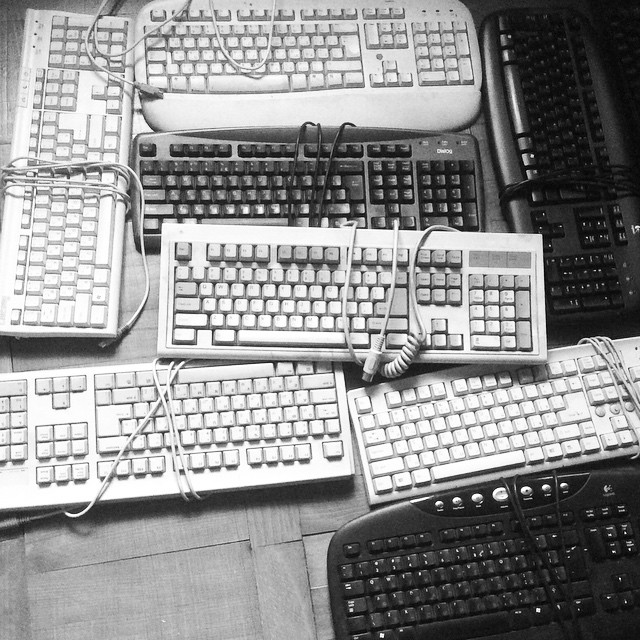The image is an overhead view of a collection of desktop computer keyboards arranged on a gray, tiled floor. There are eight keyboards in total, five of which are white and three black. Each keyboard features a numerical keypad and an F-row at the top. The cords of the keyboards are twisted around them for security. The keyboards occupy most of the frame, except for the bottom left corner where the gray floor is visible. One of the keyboards is notably positioned on top of another, adding a slight dimension to the otherwise flat arrangement of the keyboards. The photo captures the textures and details of these old computer peripherals in a clear, traditional black and white style.